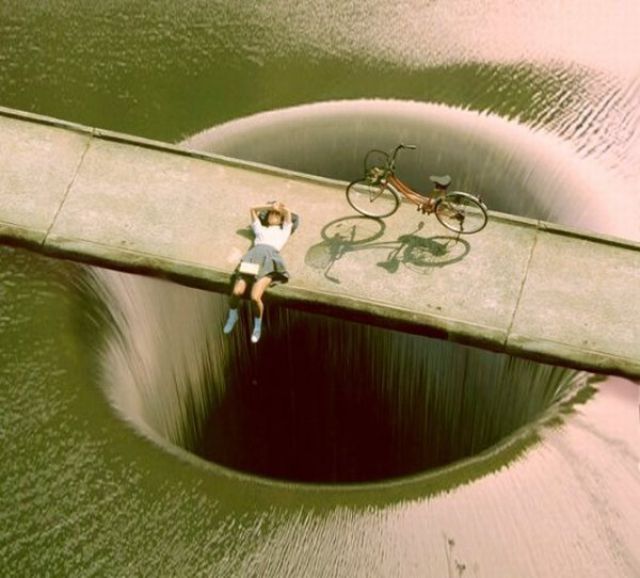In this vintage-tinted image, which exudes a subtle yellow hue, we see a surreal and slightly ominous scene of a massive body of green-hued water with a gaping, circular hole at its center, where the water is dramatically draining away. Spanning across this seemingly bottomless chasm is a concrete walkway, devoid of any railings, and featuring a pronounced lip on both sides. This cement path, gray and stark, emphasizes the precariousness of the situation.

A young girl is lying on this walkway, her body oriented along its length. She is wearing white shoes and white socks, paired with a white blouse and a pleated gray skirt. Her legs dangle perilously over the edge of the walkway from the knees down, highlighting the potential danger below. Resting on her lap appears to be a book, and she has raised her arms, placing her forearms across her forehead in a relaxed pose, perhaps to shield her eyes from the sun or sky above. Underneath her head, there is an item, possibly a gray blazer or a backpack, serving as a makeshift cushion.

To her left is a red bicycle with black handlebars and a black seat, standing upright with the help of its kickstand, which casts a distinct shadow onto the walkway. The tension between the serene appearance of the girl and the perilous abyss below adds a layer of mystery, suggesting a photoshopped nature to the image, or perhaps simply an artistic, yet eerie, creation.